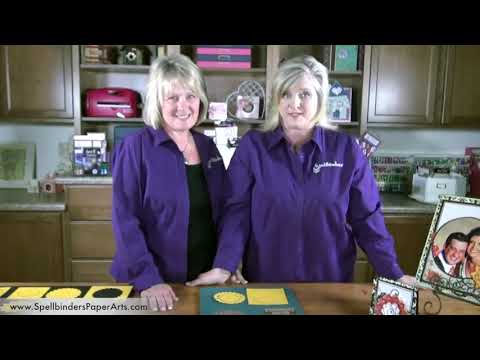This screen grab from a YouTube video features two women in a kitchen setting, likely discussing scrapbooking under the banner of Spellbinders Paper Arts, as indicated by the caption at the bottom. The women, identified as Stacey Caron and Kim Hupke, are both wearing purple jackets adorned with a logo, with Stacey's jacket worn over a black top. Their light blonde hair appears dyed, and they share similar features, though they seem more like colleagues than family, given their different last names. They stand behind a wooden kitchen counter, possibly an island, with brown wooden cabinets and shelves filled with various supplies and appliances in the background. To the bottom right, family photos in frames add a touch of personal decor to the scene. The atmosphere is casual and homely, suggesting an instructional and friendly demonstration.